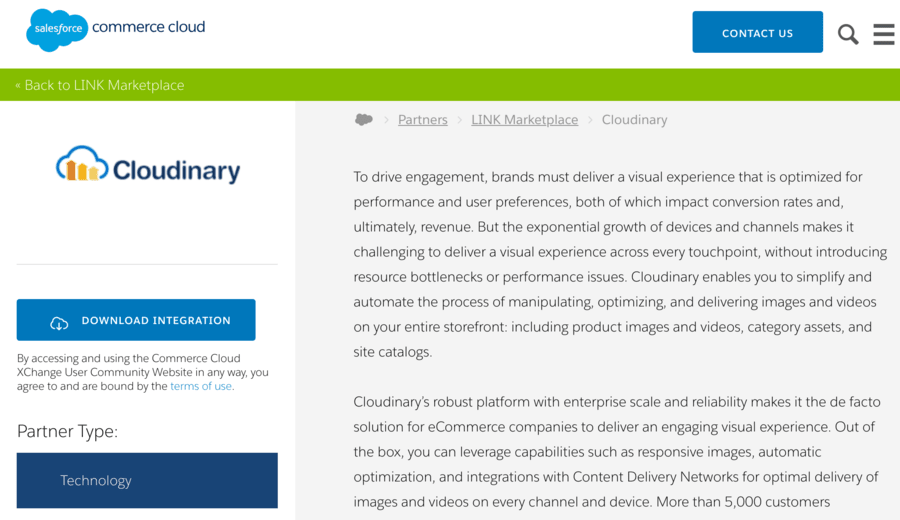The top left section of the image features the Salesforce Commerce Cloud logo alongside a blue rectangle labeled "Content Desk." A magnifying glass icon and a hamburger menu are also visible. A green label reading "Back to Link Marketplace" is situated nearby. The upper portion of the image displays the Cloudinary logo.

In the bottom left corner, the image highlights clear online integration, showcasing the use of the Commerce Cloud Exchange User Community website. It notes the binding terms of use and mentions the partner type marked by a blue rectangle labeled "Technology."

Prominent elements are the text indicating the role of Cloudinary in driving engagement by delivering a visual experience optimized for performance and user preferences, both crucial for conversion rates and revenue. However, the growing array of devices and channels complicates this delivery without causing research bottlenecks or performance issues.

Cloudinary simplifies and automates image and video manipulation, optimization, and delivery across storefronts, including product images, videos, category assets, and site catalogs. It stands out as a robust, enterprise-scale platform designed to enhance customer engagement through features like responsive images, automatic optimization, and seamless integration with content delivery networks. This ensures optimal delivery of images and videos across every channel and device, serving more than 5,000 customers. The image is slightly grainy.